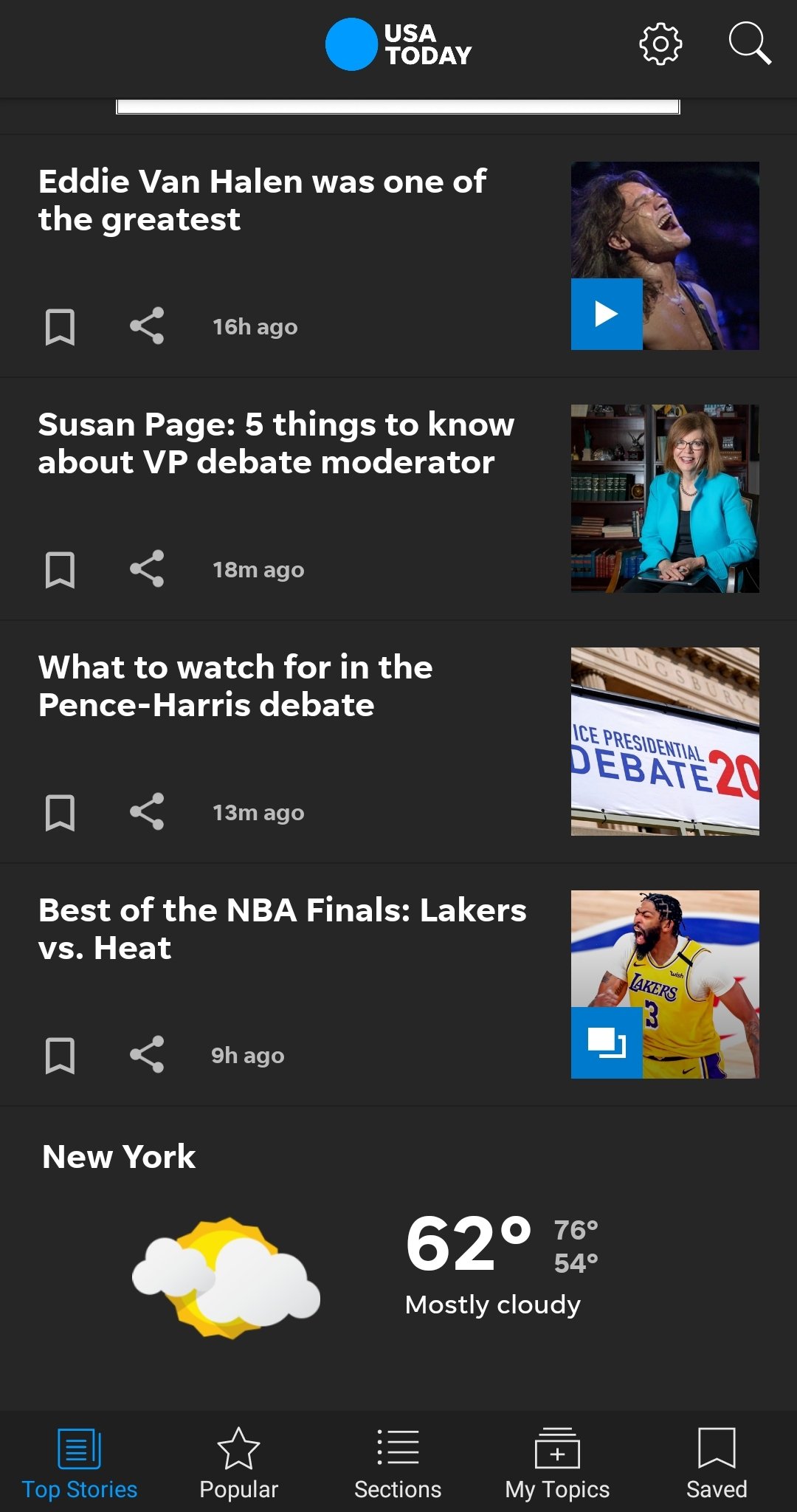This screenshot captures a mobile app displaying news and weather information, featuring a sleek and organized design. 

At the top center, the app has a dark gray background with the text "USA" on the first line and "TODAY" on the second, both in all caps and white font. To the left of this title, a vibrant blue circle stands out, while to the right, spaced out with some negative space, sit a white cog icon and a white magnifying glass icon.

Below this header, prominently in the center of the page, a thin white bar with a light gray outline is displayed, likely for search or input purposes.

Further down, articles are neatly arranged in sections separated by thin black lines. Each section features large white text in the top left corner indicating the article's title, while a square image is positioned to the right. At the bottom left of each section, there is a white bookmark icon followed by a white share icon and a small line of white text detailing the publication time. The titles and publication times of the articles are as follows:
1. "Eddie Van Halen was one of the greatest," published 16 hours ago.
2. "Susan Page: Five Things to Know About VP Debate Moderator," followed by "What to Watch for in Pence-Harris Debate," both under the same section, published 18 minutes ago.
3. "Best of the NBA Finals: Lakers vs. Heat," published 13 minutes ago.

Beneath these articles, a larger weather information section is displayed with a dark gray background. In the top left corner, the text "New York" is written in white. Slightly down and to the right, there is a cartoon-style icon of a yellow sun with an orange rim, partially obscured by a white cloud on its right side and a smaller gray cloud on the top left, casting a shadow across the sun. To the right of this weather icon, large white text indicates the temperature, "62 degrees."

This descriptive and detailed caption provides a clear and vivid depiction of the app's interface, its organized layout, and the information conveyed therein.